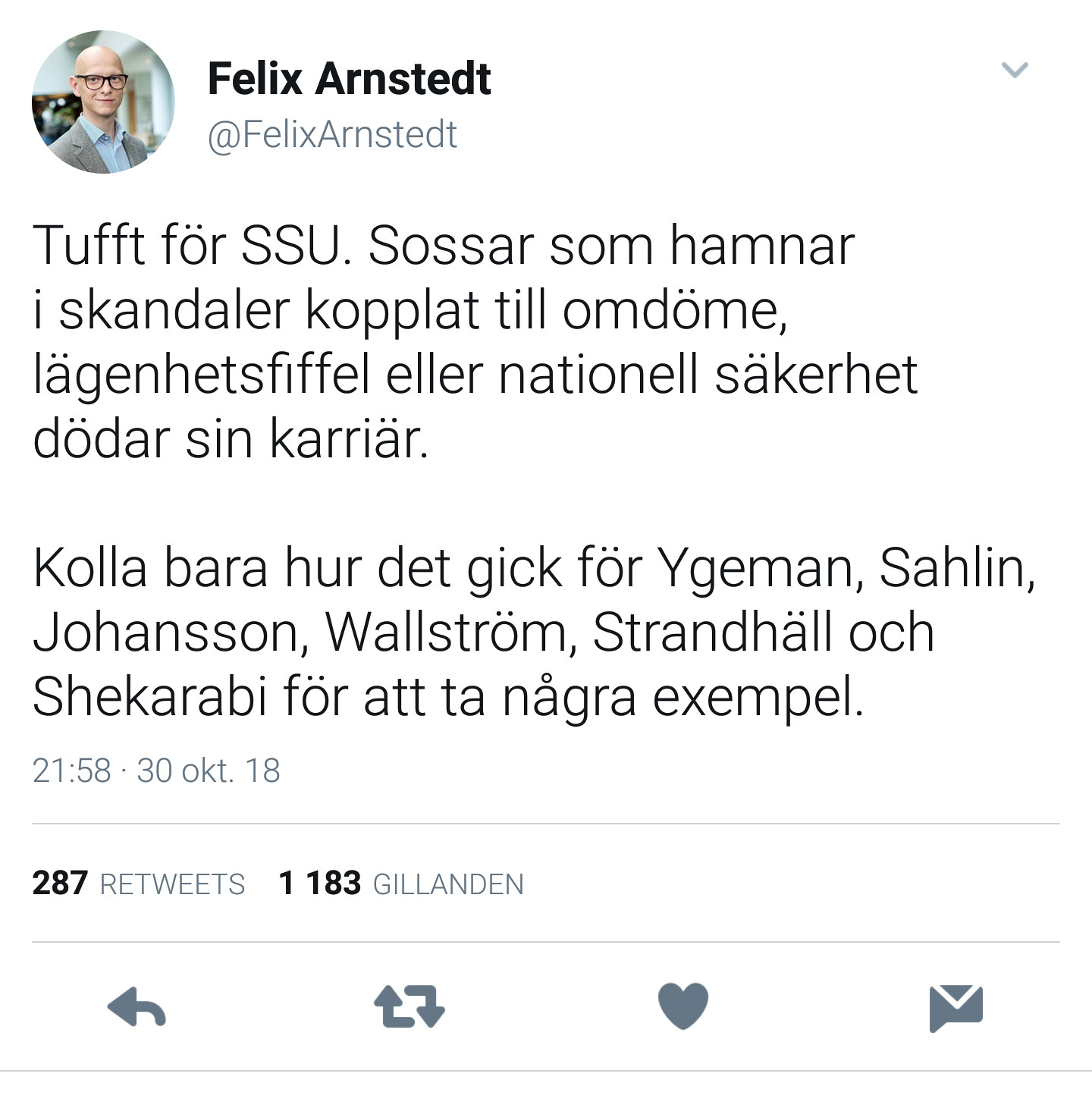This image is a screenshot of a tweet with a plain white background, seemingly taken from a website page. In the upper left-hand corner, there is a circular headshot of a bald Caucasian man wearing thick black glasses, a light gray dress jacket, and a blue collared shirt. To the right of the headshot, in bold black print, it says "Felix Arnstedt." Below his name, in lighter blue print, is his handle "@FelixArnstedt." 

The tweet itself is in a foreign language, likely German or Scandinavian, and discusses topics related to career-damaging scandals among certain individuals within national security and other high-profile positions. It mentions names like Y-G-E-M-A-N, Salin, Johansson, Wahlstrom, Strandhal, and Shekarabi as examples. 

Below the tweet text, in light gray print, is the timestamp, "21:58, 30 OKT" (October 30), and it notes that the tweet has "287 retweets" and "1,183 likes" (gillendin). At the bottom, there is a gray arrow pointing to the left, two arrows indicating refresh, a gray heart, and a gray envelope icon.